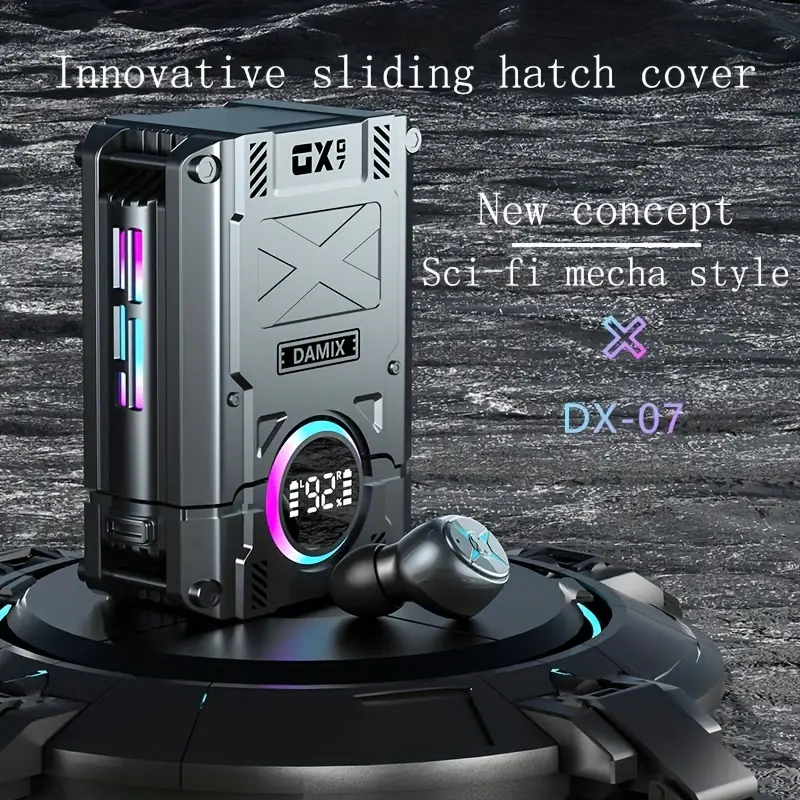Set against a black, grayish, and white background that evokes the surface of a distant planet, this advertisement showcases an innovative sliding hatch cover, presented in prominent white text. The highlighted product, featuring a new concept in a sci-fi mecha style, displays a gradient X transitioning from blue to purple to pink, followed by the model number DX-07 in similar hues.

The focal point of the image is a sophisticated device, possibly a case or charging unit for Bluetooth earphones. This square, metallic black case sits atop a round base and is equipped with four legs, giving it a futuristic and sturdy appearance. The case features a blue X on its side and is engraved with GX and G7. Centrally located on the box is the name DAMIX.

A significant feature of the case is the power gauge prominently displayed on the front, reading 92%, flanked by battery symbols labeled L (left) and R (right), indicating the charge levels for left and right earphones respectively. Surrounding the gauge are colors of purple, white, and blue lights.

In front of this box lies one of the showcased Bluetooth earphones, also black with a cushioned end and adorned with a cyan-colored X and a black circle at its center. The advertisement effectively combines a futuristic aesthetic with practical features, appealing to fans of high-tech design.